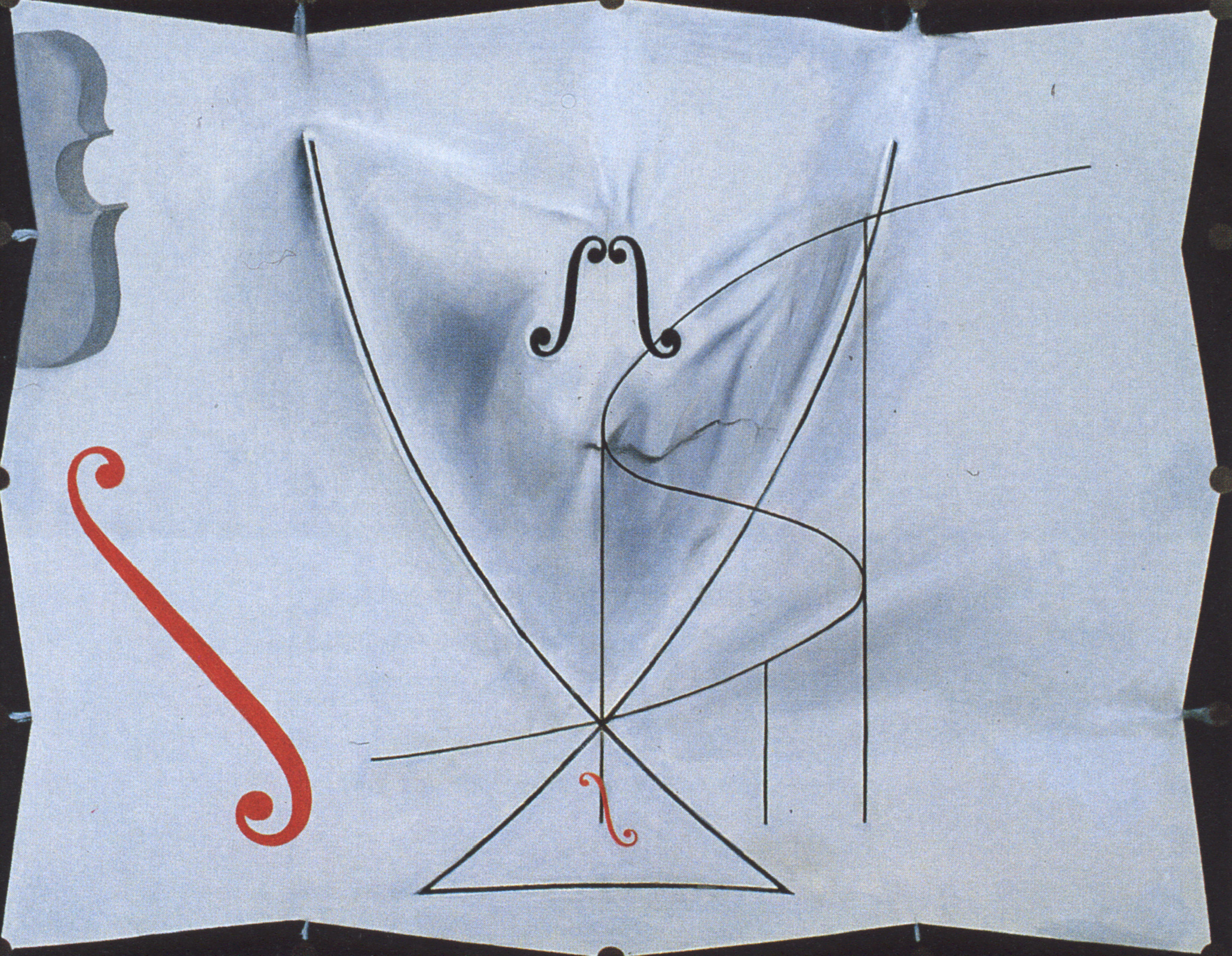The image is an abstract, intellectual art piece depicted on a sheet of white paper with a predominant black and white color scheme, accented by red and gray elements. Centered on the paper, various lines trace geometric shapes and abstract figures. Notably, there are representations of the S-holes from a cello or violin: two black S-holes occupy the middle portion, while a larger red S-hole is situated at the bottom left corner and a smaller red S-hole appears at the bottom. In the upper left quadrant, there is the gray outline of a cello or violin body, partially forming a face-like image with a discernible nose and line resembling a mouth. Additional long lines traverse the image both horizontally and vertically, adding to its complexity. The artwork is framed by a black border, uniting the abstract forms into a cohesive, thought-provoking composition.